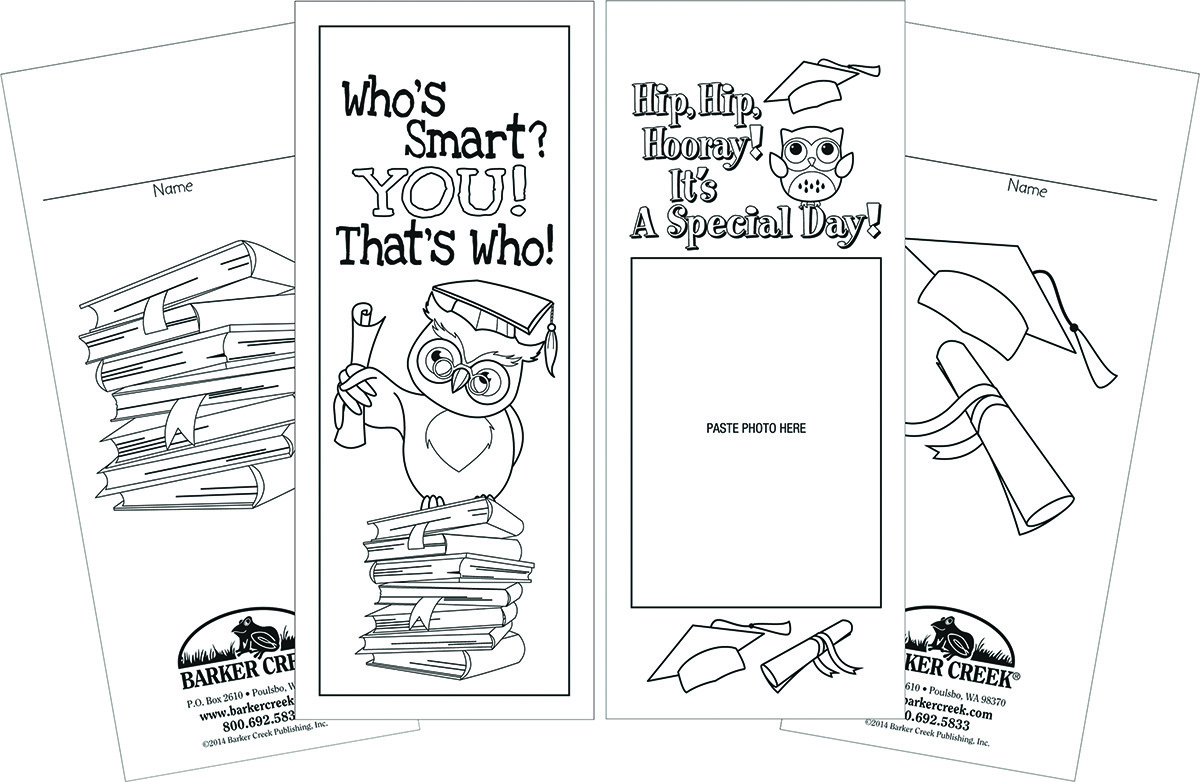The image is of a black and white educational brochure from Barker Creek, featuring detailed line drawings and various celebratory themes. The brochure consists of multiple pages, with no border around the image. On the leftmost page, it says 'Name' with an underline and displays the Barker Creek logo along with a telephone number, P.O. box, and email address. There is a stack of books, two of which have bookmarks.

The next page features bold black lettering that reads, "Who is smart? You, that's who." It includes an intricate line drawing of an owl wearing a mortarboard, perched on a stack of seven books, and holding a scrolled diploma. The owl wears reading glasses and the mortarboard has a feather on it.

The following page announces "Hip hip hooray, it's a special day" in bold black letters and depicts the same owl tossing his mortarboard into the air. Below this cheerful illustration, there's a designated space labeled "Paste photo here," adorned with images of a graduation cap and a scrolled diploma.

On the rightmost page, similar to the leftmost one, it says 'Name' with an underline and includes the same large images of a mortarboard and a scrolled diploma, alongside the Barker Creek logo, contact information, and the logo featuring a frog.